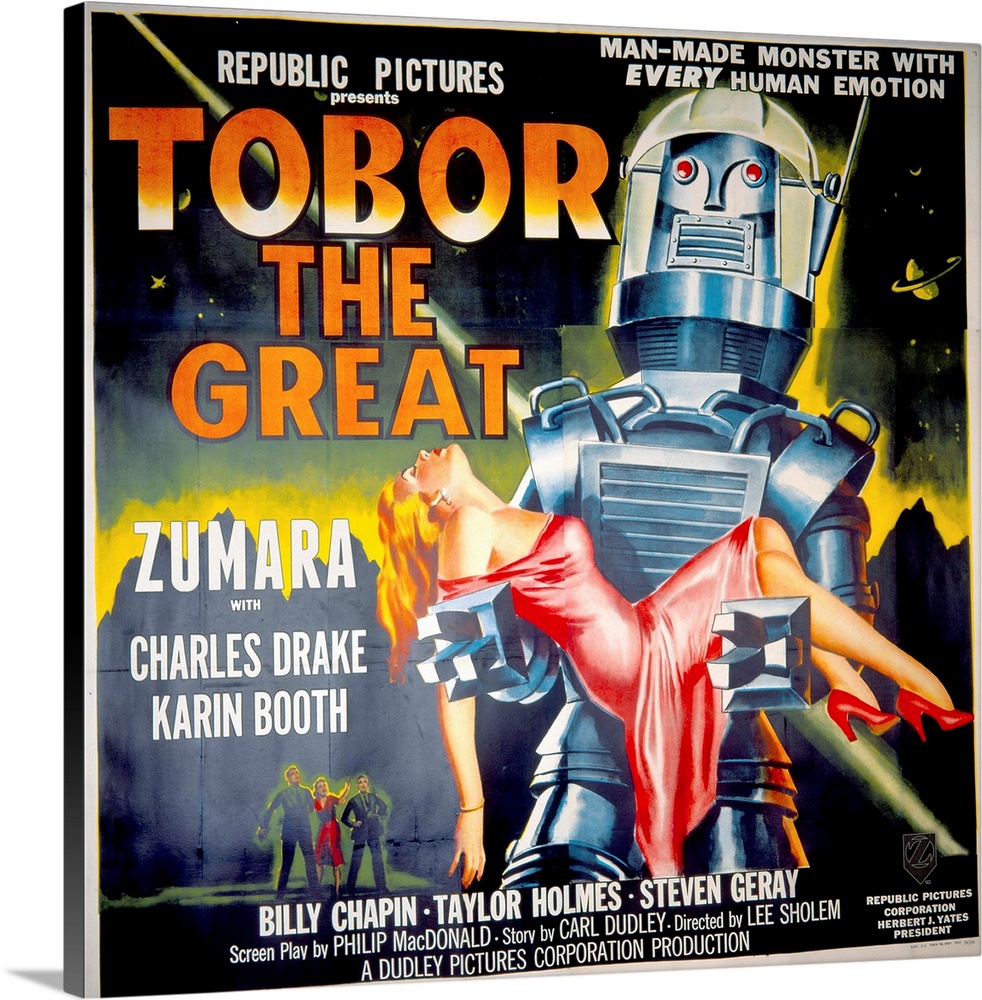The image is a striking movie poster from Republic Pictures for the film "Tobor the Great." Dominating the scene is a large robot with red eyes, crafted from bluish metal, giving a human-like appearance with two arms and two legs. The robot's mouth is a rectangular slot with rivets, and it wears a helmet. In its arms, the robot holds an unconscious beautiful woman dressed in a strapless red dress and matching red heels. To the side of the robot, a depiction of the planet Saturn is visible against the predominantly dark background. The poster also features distant small figures, hinting at additional characters.

The movie's title, "Tobor the Great," is prominently displayed in big orange letters on a black background. The tagline reads, "Man-made monster with every human emotion." Cast members listed include Billy Chapin, Taylor Holmes, and Stephen Geary, with further mention of stars Zumara, Charles Drake, and Karen Booth. The Republic Pictures Corporation logo is positioned in the lower right corner of the poster. Overall, the poster evokes a classic science fiction feel with an intriguing mix of human and robotic elements.